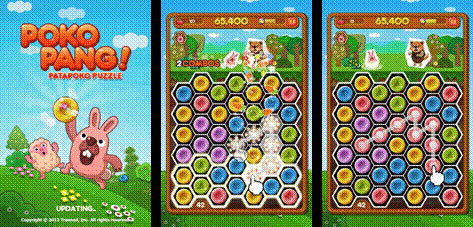This image collage features three distinct photographs, each contributing to an overarching theme centered around a game. The first photograph depicts a scene reminiscent of a jigsaw puzzle box, identified as "Poco Pong" with the subtitle "Patapoco Puzzle." In this setting, a whimsical cartoon bunny rabbit with prominent, elongated white teeth is portrayed scampering across a verdant hillside. He appears to be playfully chasing a baby sheep amidst a picturesque landscape adorned with blooming flowers and lush green trees in the background.

The second photograph transitions the viewer into the gameplay itself. Here, the screen is teeming with a multitude of vibrant, circular discs in a palette of colors including green, yellow, pink, blue, and purple. A small, white hand is seen actively pressing one of these colorful discs. Some of the discs appear illuminated, glowing with a white hue, indicating interaction or selection.

In the third photograph, the gameplay screen is depicted again, maintaining the same lively arrangement of colored discs. This time, the image zooms in on the action, showing the white hand pressing one of the discs. A noticeable white line forms a connecting pattern between several of the discs, suggesting the progress or strategy within the game.

Overall, the collage captures the essence of the game, juxtaposing a playful cartoon scenario with dynamic, interactive gameplay elements.